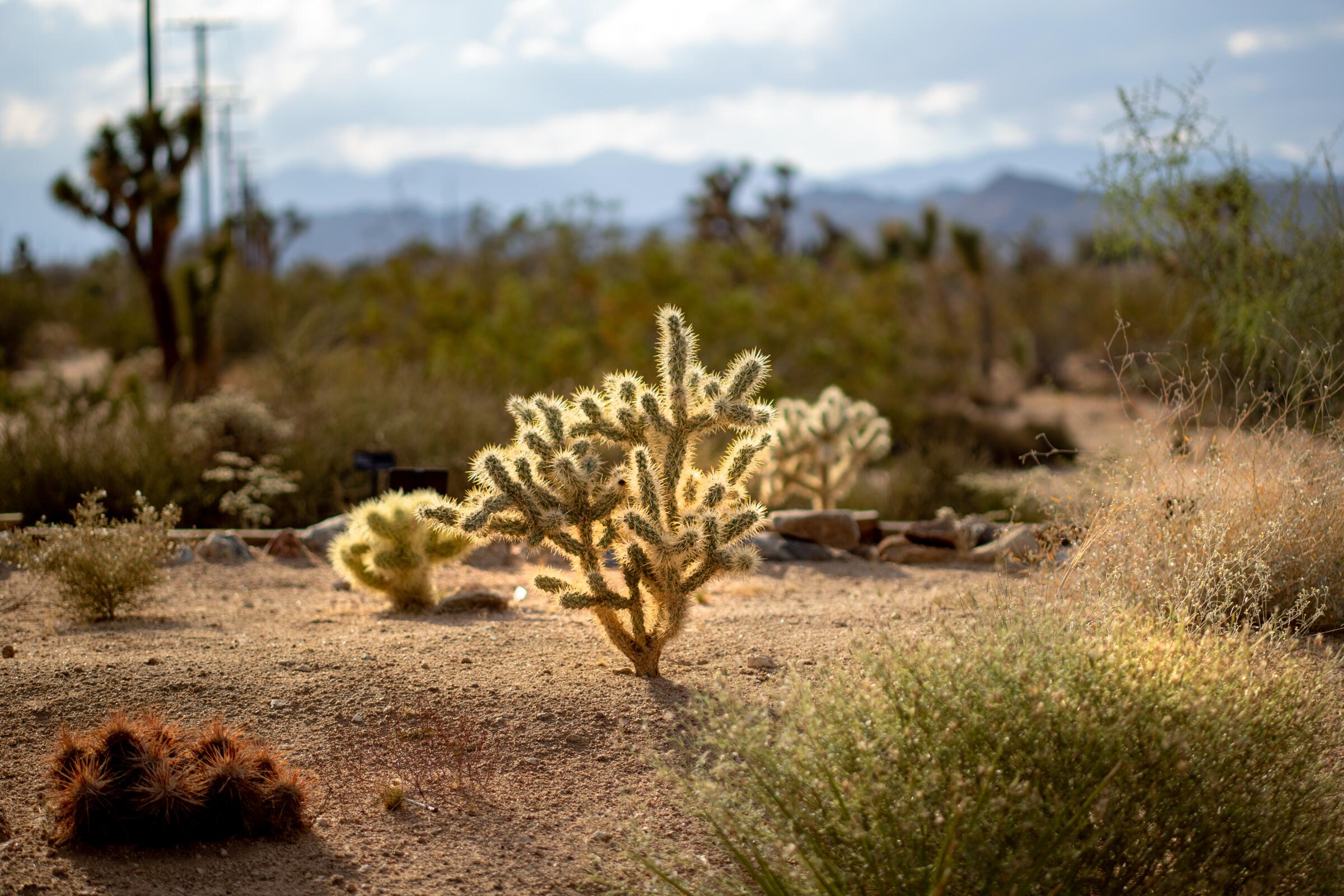This close-up image captures a desert scene with a small, bush-like cactus plant as the central focus. The plant, emerging from light brown, dusty sand, features a short stem with multiple offshoots that fan out horizontally before curving upwards. Each offshoot is adorned with green, cylindrical segments covered in light green fuzz and yellow spines, giving a prickly appearance. The background, though blurred, reveals a light blue daytime sky dotted with puffy white and gray clouds. You can faintly see dark gray mountains and hills along the horizon, as well as some tall telephone poles on the left side, indicating it's not an entirely remote area. The surrounding vegetation consists of dark green grass and taller shrubs, emphasizing the arid yet life-sustaining environment.